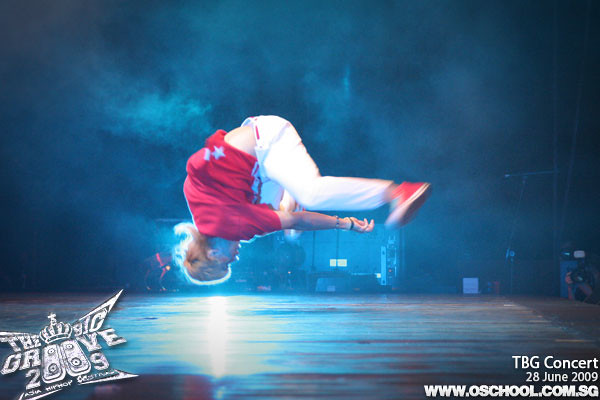The photo captures a dynamic moment of a dancer performing an acrobatic move in mid-air, seemingly caught in the middle of a forward somersault or flip with his head pointing downward and feet up in the air. The dancer, who has blonde hair, is dressed in a red shirt, white pants, and red shoes. He appears to be on a stage, identifiable by the brown wooden surface partially visible near the bottom of the image. The stage is bathed in blue light, which, along with the surrounding smoke also tinged blue, creates a dramatic atmospheric effect. In the lower left corner, the text "The Big Groove 2009" along with a crown symbol is clearly visible. Meanwhile, the lower right corner features the text "TBG Concert 28 June 2009" followed by the website "www.oschool.com.sg." The overall scene suggests a well-lit performance in a dark, indoor setting, emphasizing the skill and motion of the dancer.